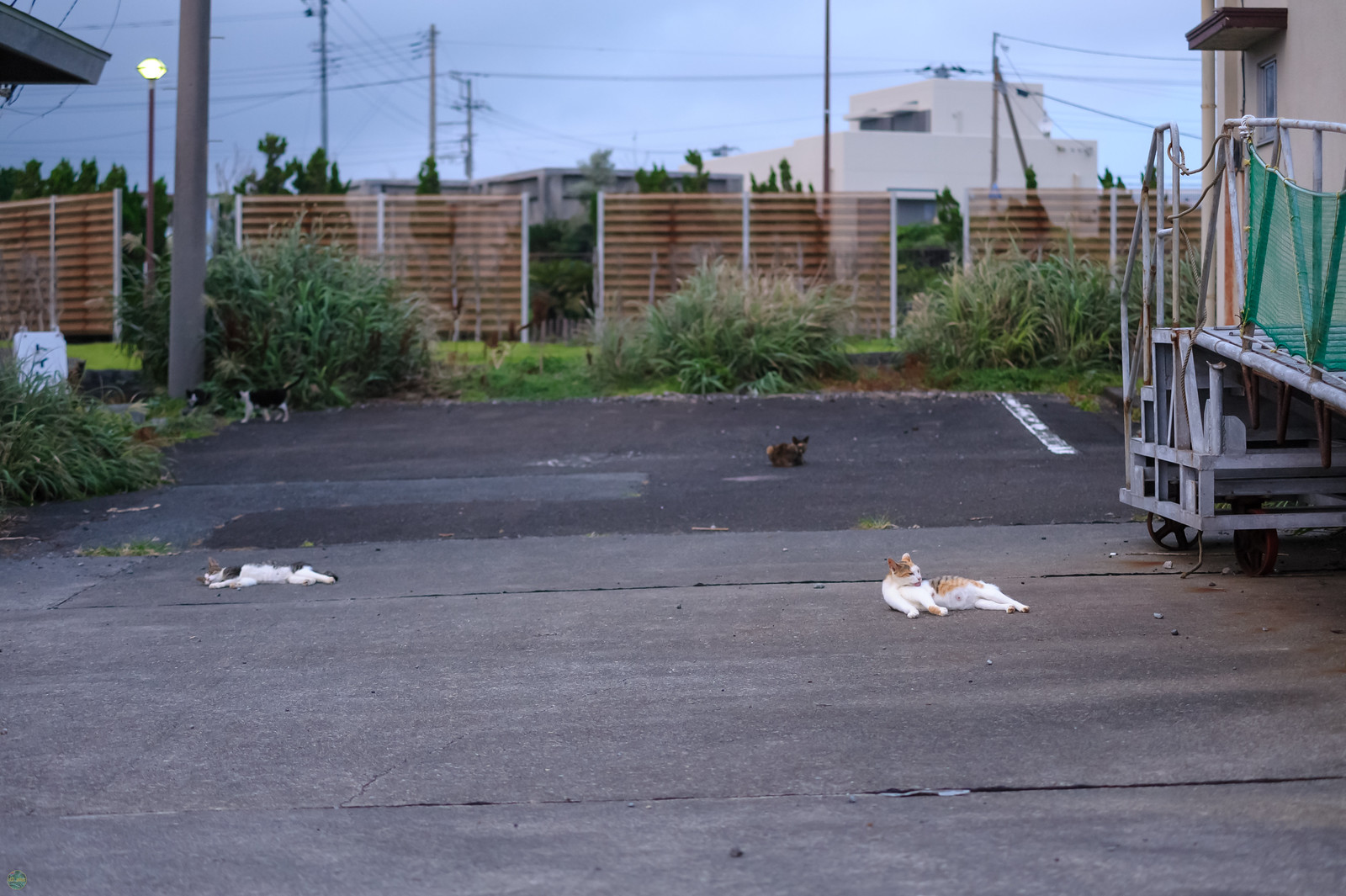This is a detailed landscape photograph in color depicting an outdoor scene, possibly a parking lot, with a gray asphalt surface. Prominent in the foreground are three small cats. The first cat on the left has black and white markings and is laying on its belly. The second cat, slightly to the right, is orange and white and is lying on its side with its legs stretched out. A third animal, likely a small dog, can be seen farther in the background standing on all fours with its head facing the camera. 

On the right side of the image, a silver metallic ramp leads up to a white building with a small window. There is also some green netting or a shade cloth hanging from the side of the ramp. To the back of the lot, there are tall grasses with seed heads, some green shrubbery, and a brown wooden fence. Beyond the fence, there are a few higher buildings, one of which has a gray color, and a series of telephone poles with overhead wires. A streetlight is visible on the left side of the background. The sky is a light blue, indicating daytime, but the exact time could be dusk or dawn given the streetlight's presence.